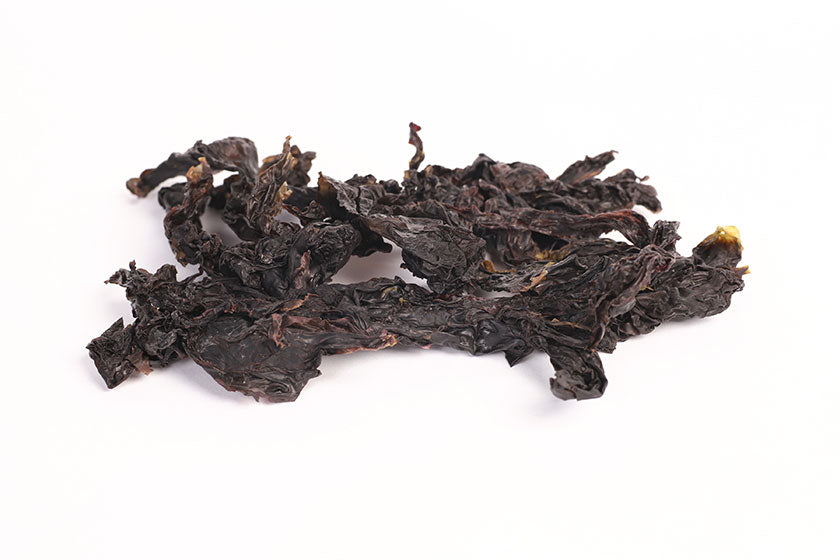In the center of the stark white background lies a dark, twisted mass that dominates the image. This mysterious object appears charred or burnt, possibly resembling a piece of seaweed, plant matter, or even crumpled paper. Its intricate folds and twisted structure suggest it was once longer but has been shriveled and contorted into an oval shape. The predominant color is a deep, almost black brown, with varying shades of medium brown woven throughout. Tiny edges along the mass reveal hints of an orange or yellow hue, lending a striking contrast. This object lies mangled, with parts sticking up and detailed textures that imply it has been dried out or subjected to fire, casting shadows that hint at an external light source. The entire image focuses on this mysterious, centrally positioned, and thoroughly burnt material.